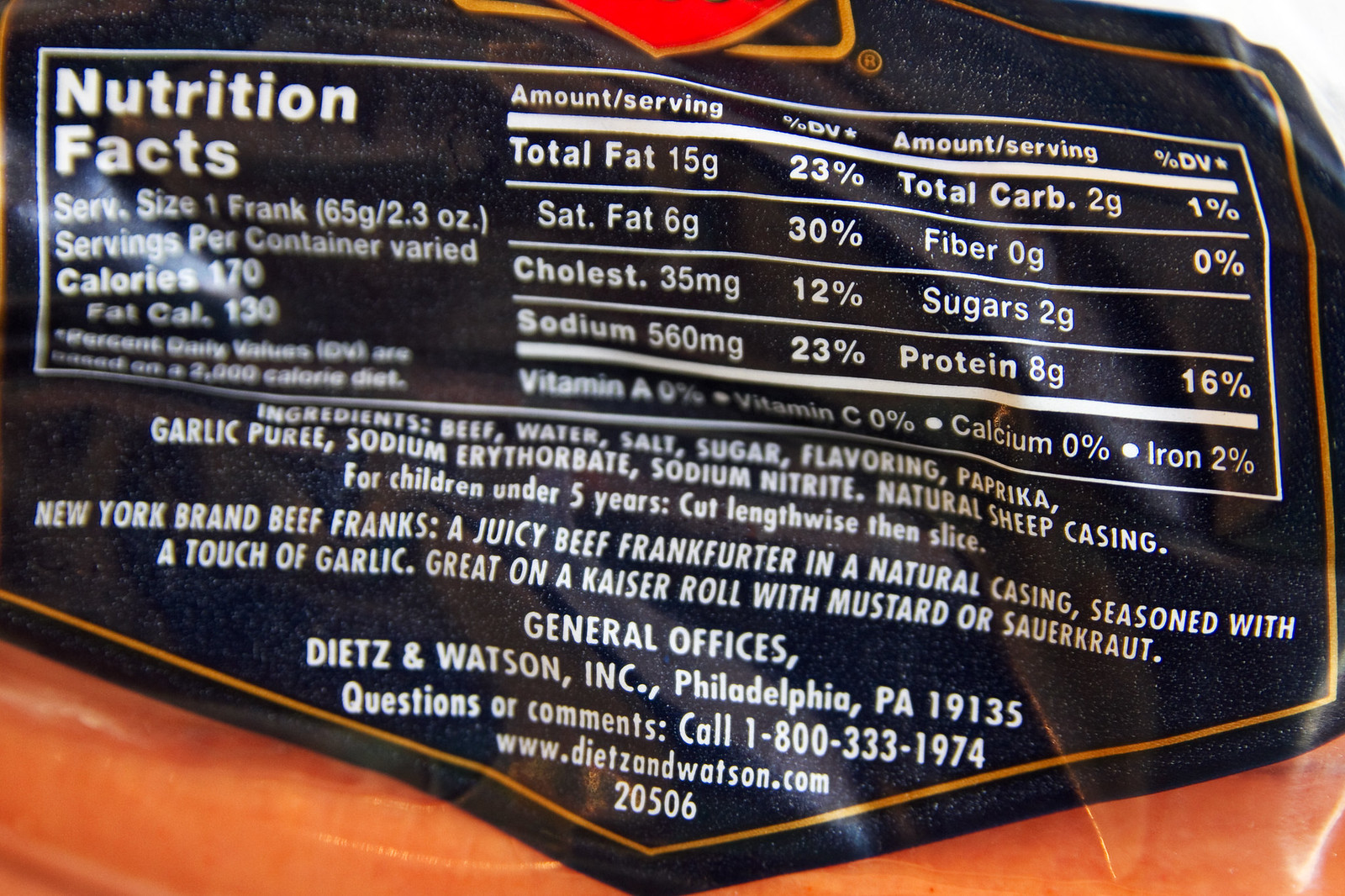This image features the back of a product showcasing its nutritional facts label. The item, identified as "New York Ground Beef Franks," provides detailed serving information: one frank weighing 65 grams or 2.3 ounces. Each serving contains 170 calories, including 130 calories from fat. The label lists total fat at 15 grams, saturated fat at 6 grams, cholesterol levels at 35 milligrams, and sodium content at 560 milligrams. Additionally, it provides nutritional content for total carbohydrates at 2 grams, dietary fiber at 0 grams, sugars at 2 grams, and protein at 8 grams. 

Below the nutritional facts, the label mentions vitamin and mineral content, including Vitamin A, Vitamin C, calcium, and iron. It also features essential consumer information and precautions, advising against consumption by children under 5 years old and suggesting that franks be cut lengthwise before slicing. 

The product is described as juicy beef frankfurters in natural casing, seasoned with a hint of garlic, and recommended for serving on a kaiser roll with mustard or sauerkraut. The label is predominantly black with white text and includes company details: Dietz and Watson Incorporated, headquartered in Philadelphia, Pennsylvania (19135). Contact information for consumer inquiries, including a phone number and website, is also provided. The bottom of the label features the number "20506," though its significance is unclear.